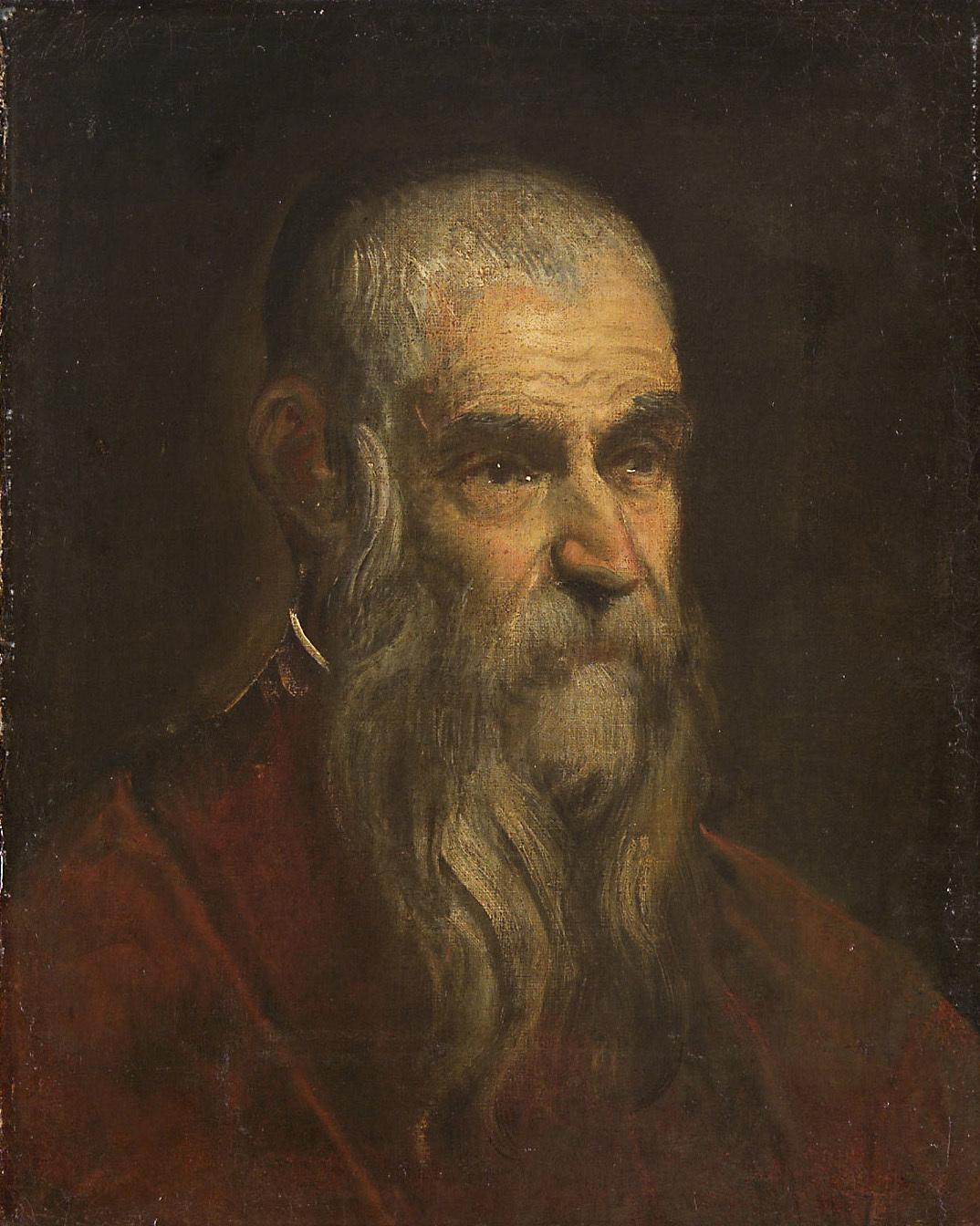This is an aged oil painting, showing signs of wear and fading, with some of the canvas fabric visible through the surface. The portrait is of an older man with fair skin, characterized by short, thinning hair on top and a long, gray beard and mustache. His bushy, dark eyebrows and prominent nose are notable features, along with a wrinkled forehead. The man is dressed in a dark reddish cloak or jacket that reaches up to his neck, covering his shoulders and chest. He is looking slightly to the right, offering a partial side view of his face, which appears to have teary, brown eyes. The background is a very dark color, predominantly a dark brown or gray with a slightly lighter area giving a subtle halo effect around his head and neck.